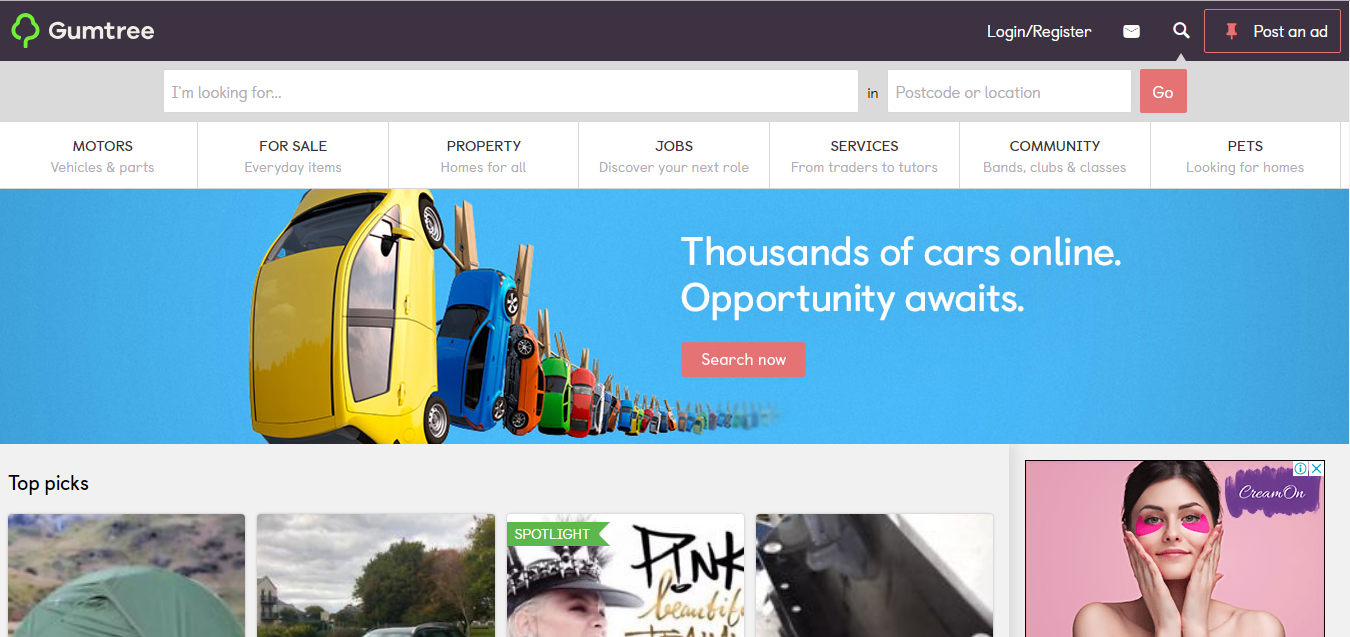This is a detailed screenshot from the Gumtree website. At the very top, there is a black navigation bar. Positioned in the upper left corner of this bar is the Gumtree logo, featuring a simple green tree icon next to the white text "Gumtree." On the right side of this bar, there are options for users to log in or register, along with a button labeled "Post an ad."

Just below this navigation bar, there is a primary search area. The left search box has placeholder text that reads "I'm looking for," while the adjacent search box says "postcode or location." An orange "Go" button is situated next to the search fields.

Directly underneath this search area, there is a set of categorized options, including "Motors for Sale," "Property," "Jobs," "Services," "Community," and "Pets."

The main portion of the screenshot is dominated by a large, eye-catching banner. The background of the banner depicts a blue sky with a laundry line. Uniquely, various colorful cars are hanging from the laundry line by clothespins. Adjacent to the hanging cars, the banner's text reads, "Thousands of cars online. Opportunity awaits." A vibrant red "Search Now" button is prominently displayed next to this text.